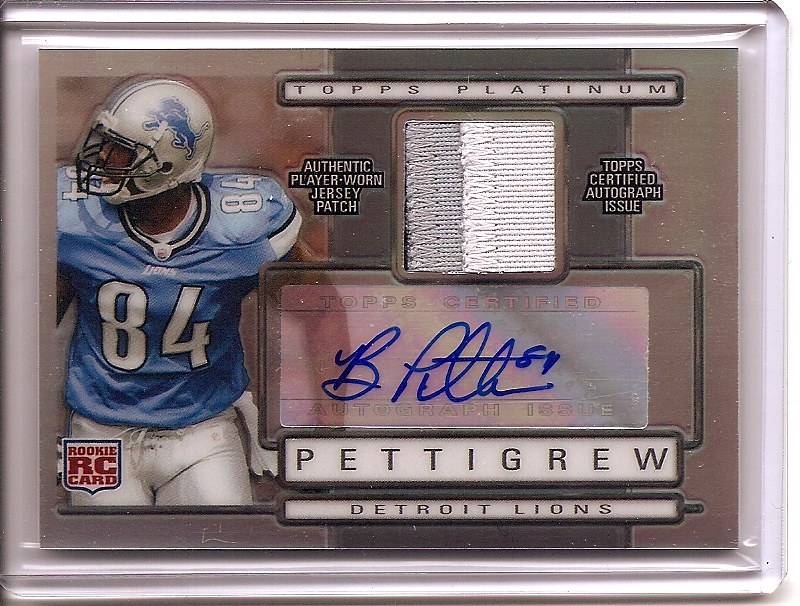This is a highly detailed and embossed Topps Platinum football trading card of Detroit Lions' player, number 84, Pettigrew. The card, which is encased in a protective card holder, features a silver frame and showcases a light blue jersey-wearing Pettigrew on the left side, complete with a traditional silver helmet adorned with the blue lion emblem. The card's overall design includes a small square cutout displaying an authentic player-worn jersey patch, labeled on the left as "Authentic Player Worn Jersey Patch". On the right side, it prominently reads "Topps Certified Autograph Issue" with a corresponding silver foil badge and Pettigrew’s autograph in blue sharpie above it. Additionally, the card identifies it as a "Rookie RC Card" in a red text bubble located at the bottom left corner. The player's name, "Pettigrew," and his team, "Detroit Lions," are clearly printed beneath the autograph section. The entire card, including the player's outline, is embossed, adding to its premium feel.